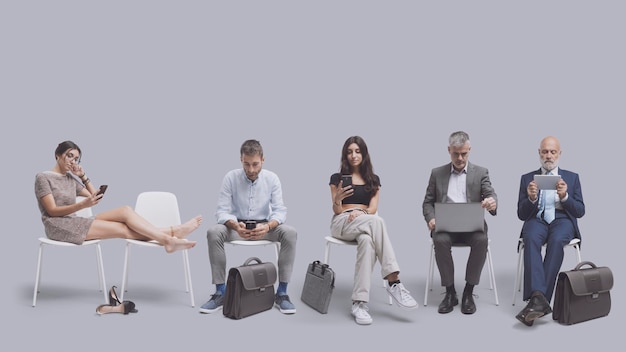The photograph captures five people sitting on six white plastic chairs arranged in a row against a plain gray backdrop. Each individual is absorbed in their own electronic device, giving the image a staged and modern feel.

Starting from the left, a woman is occupying the first chair and has her legs stretched out onto the second chair. She is barefoot, with her shoes placed on the ground between the two chairs. She wears a short-sleeved, beige-colored dress that ends at her upper thighs. Her dark brown hair is pulled up at the back, and she is engrossed in her cell phone, which she holds in her right hand.

To her right, a man is seated on the third chair, with his legs slightly spread apart and both hands on his cell phone. He wears a light blue button-down shirt and gray trousers, accompanied by casual light blue shoes. A soft leather briefcase is positioned between his feet, directly beneath his seat.

Next to him, occupying the fourth chair, is another woman. She sports a dark top that exposes her midriff, paired with light-colored blue jeans and white high-heeled shoes. Her long, dark hair cascades over her shoulders, and she is also fixated on her cell phone held in her right hand. Her right leg is crossed over her left, and a thin briefcase leans against her chair's right leg.

In the fifth chair sits a man dressed in a light gray suit without a tie, his collar open for a more relaxed look. He has short, graying hair and dark shoes. He is focused on a silver laptop resting on his lap, his hands positioned on its upper and lower portions.

Finally, on the far right, a man in a dark blue suit and a light blue tie occupies the sixth chair. He is bald with a gray beard and mustache, resembling Michael Stipe. His legs are crossed, and he is intently looking at a small, slate-colored tablet held horizontally in his hands. A large leather briefcase, matching the one owned by the man on the third chair, sits to his left.

Overall, the image conveys a sense of individual disconnection amidst a shared, staged setting.